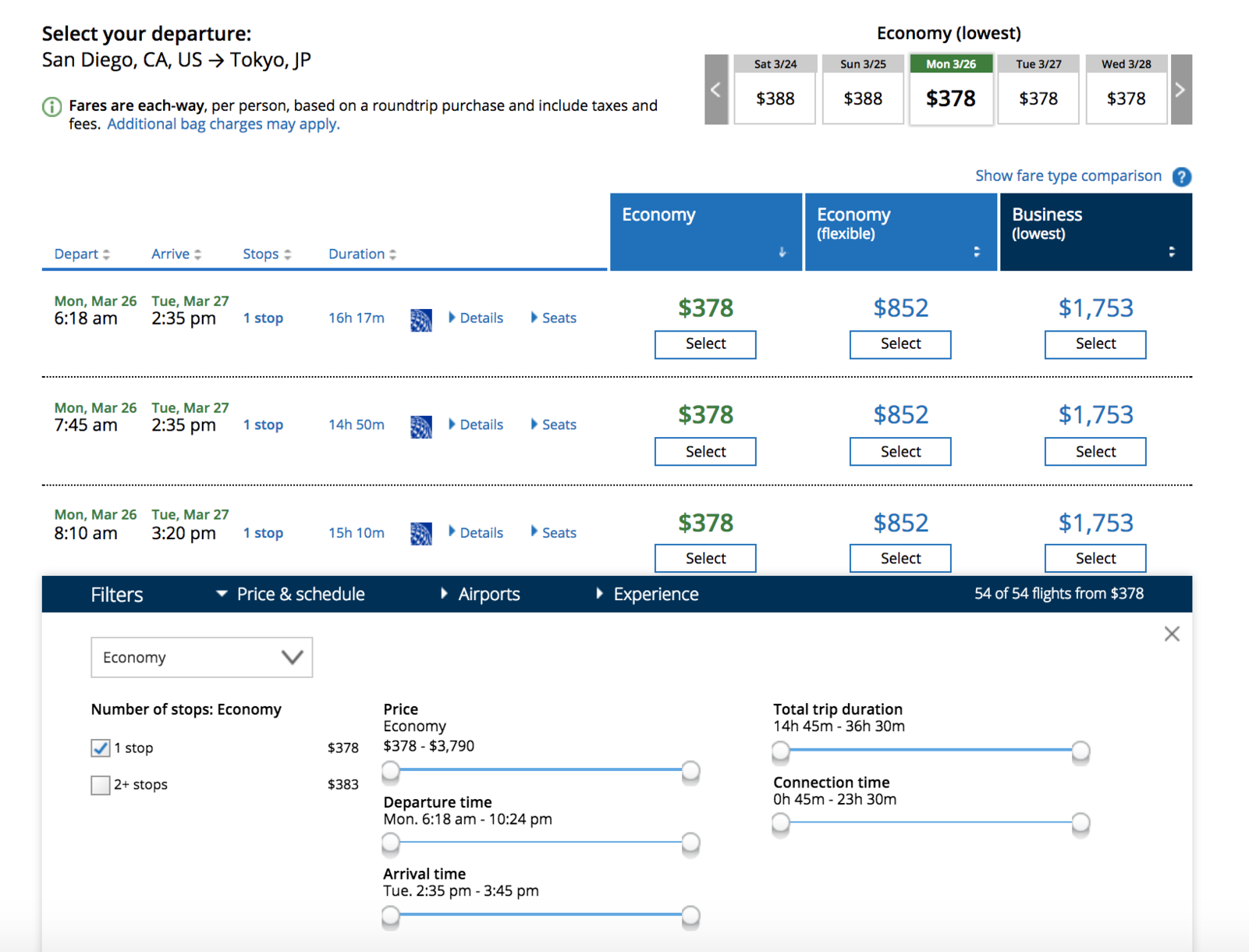Here is the cleaned-up and detailed caption:

---

**Flight Schedule for a One-Way Trip from San Diego, California to Tokyo, Japan**

Travel Date: Monday, March 26th 

**Option 1:**
- **Departure:** 6:18 a.m. 
- **Arrival in Tokyo:** 2:35 p.m. (the next day)
- **Duration:** 16 hours and 17 minutes
- **Stops:** 1 Stop
- **Economy Class:**
  - **Standard Economy:** $378
  - **Flexible Economy:** $852
- **Business Class:**
  - **Lowest Price:** $1,753

**Option 2:**
- **Departure:** 7:45 a.m.
- **Arrival in Tokyo:** 2:35 p.m. (the next day)
- **Duration:** 14 hours and 45 minutes
- **Stops:** 1 Stop
- **Economy Class:**
  - **Standard Economy:** $378
  - **Flexible Economy:** $852
- **Business Class:**
  - **Lowest Price:** $1,753

**Additional Information:**
- Travelers opting for economy class with multiple stops will find prices starting at $383. 
- Economy class fares range from $378 to $3,790 depending on the number of stops and the flexibility of the ticket.